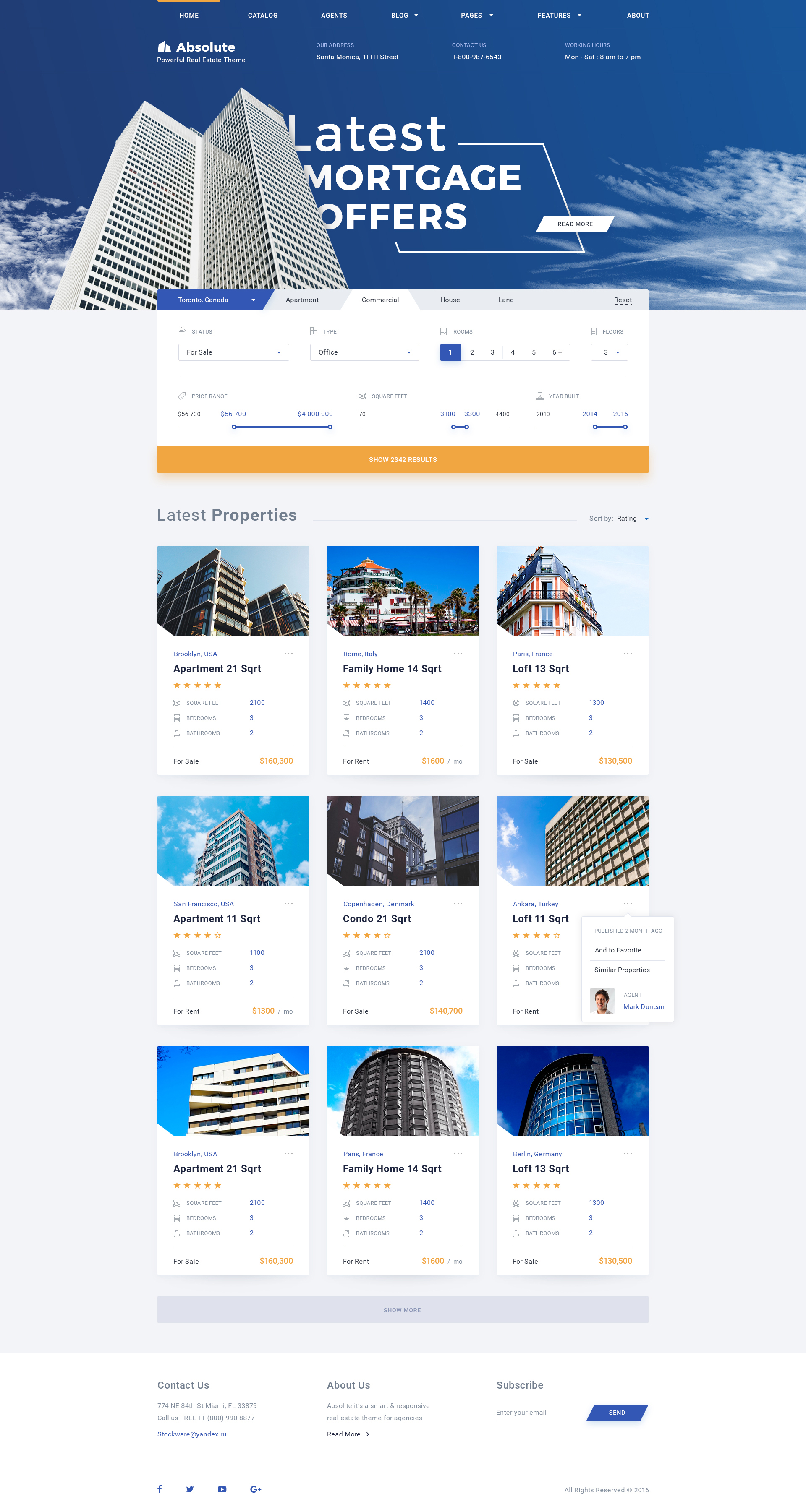The webpage being described belongs to "Latest Mortgage," prominently featuring its name "Absolute" at the top alongside the tagline "Powerful Real Estate Theme." The website header includes contact information, displaying an address at "11th Street, Santa Monica," a phone number, and operational hours from Monday to Saturday, 8 AM to 7 PM.

Below the header, the page showcases a striking image of two towering skyscrapers against a clear blue sky adorned with a few white clouds. The headline "Latest Mortgage Offers" is prominently displayed above actionable content, including a "Read More" button.

Further down, navigation tabs offer filters such as "Toronto, Canada" (highlighted in blue), "Apartment," "Commercial," "House," "Land," with an option to reset selections. The current selection features "Toronto, Canada," with a status dropdown for properties for sale and the property type marked as "Office."

Additional search parameters allow customization: room count (currently set to 1 but adjustable up to 6+), floor selection (starting at 3+), and price range (from $56,700 to $4 million). There is also an option to refine the search by square footage and year built. 

The page indicates 2042 results in an orange banner. Thumbnails of the latest properties are displayed below, each including details like apartment number, price, bedroom and bathroom count. There are a total of nine property listings visible.

At the bottom, there is a "Show More" button, further contact information, an email link for composing inquiries, an "About Us" section, and a subscription option.